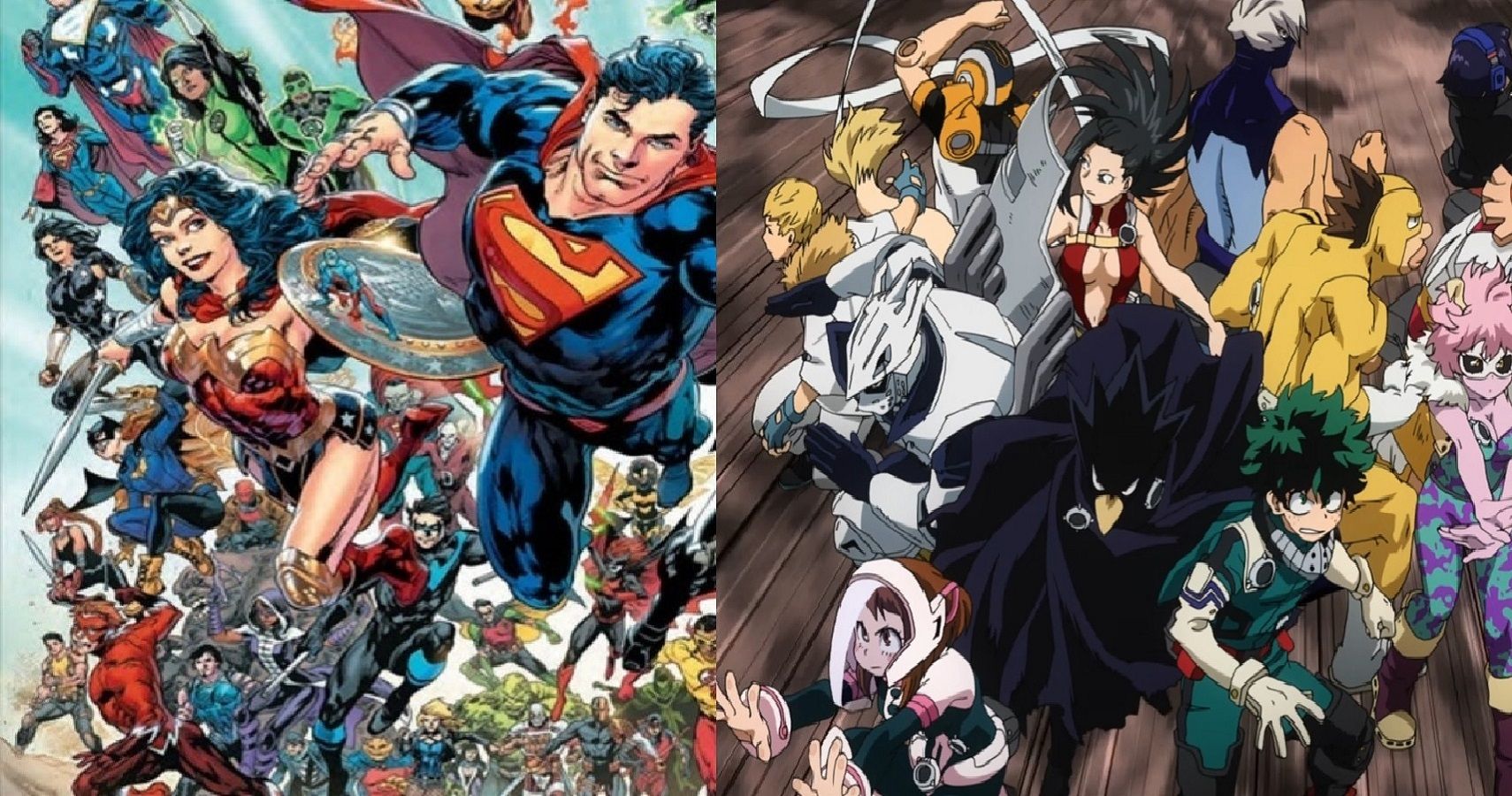The image consists of two side-by-side cartoon drawings, distinctly divided by style and character universes. The left side features iconic DC superheroes, prominently showcasing Superman and Wonder Woman, both flying towards the viewer. Superman is easily recognizable with his blue, red, and yellow costume, while Wonder Woman is situated to his left in her classic attire. Other characters such as the Flash and potentially the Hulk, although typically a Marvel character, are scattered in the background amidst a flurry of indistinct figures, all set against a vibrant backdrop with colors including blue, red, green, yellow, black, purple, and pink.

In contrast, the right side depicts a group of anime-style characters, recognizable by their Japanese manga aesthetic. The scene is set against a darker background and includes both male and female characters, some wielding weapons like swords, while one character appears to be using telekinesis. Among the anime characters, a central figure closely resembles a black bird. The color palette on this side includes darker shades with accents of black, white, green, gray, blue, red, orange, and purple.

Without any visible text in either image, the overall composition highlights a vivid juxtaposition of Western superheroes and Eastern anime characters, each side bursting with diverse colors and dynamic poses.